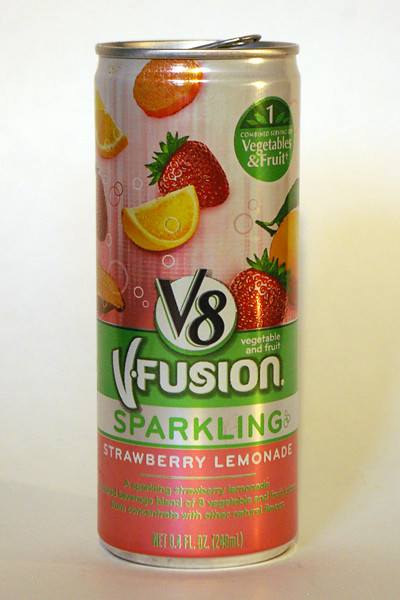This photograph captures a can of V8 V-Fusion Sparkling Strawberry Lemonade, prominently positioned against a crisp white backdrop. The setting appears to be an amateur studio with minimalistic lighting, creating subtle shadows that accentuate the contours of the can. The can features the iconic V8 logo prominently in the center, with "V-Fusion" inscribed just below it. Above the logo, small text reads "Vegetable and Fruit," emphasizing the blend's wholesome ingredients. The description continues below with "Sparkling Strawberry Lemonade," detailing the flavor. At the bottom, further text specifies it is a "Beverage blend of eight vegetable and fruit juices from concentrate with other natural flavors." The can's capacity is noted as 8.4 fluid ounces (248 milliliters). The upper section of the can is adorned with small, vibrant images of fruits and vegetables, visually reinforcing the product's natural and healthy branding.